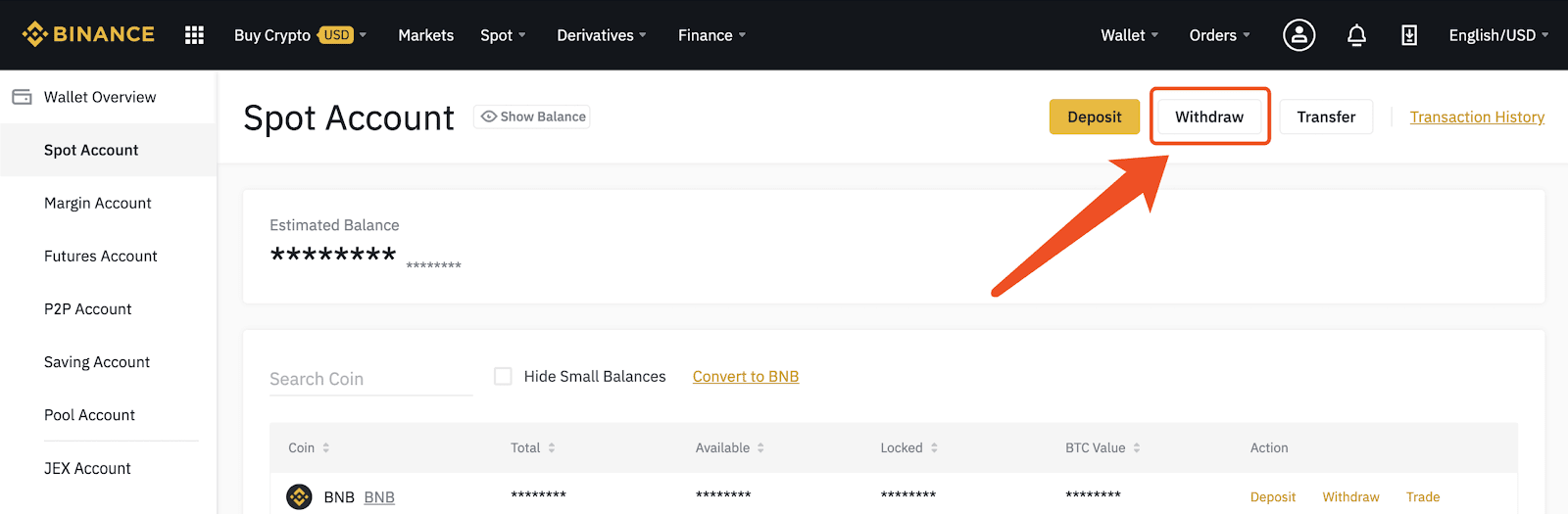### Detailed Caption:

The image showcases a screenshot of the Binance website viewed on a personal computer. The web page appears to be in the "Finance" section under the "Crypto Spot Account" view. The user has navigated to the "Withdrawal" section, but no specific transaction details are visible. 

At the top of the page, a black navigation bar features "Binance" prominently in bold letters with a yellow and black outline. Next to the logo, menu items are listed: "Buy Crypto" in yellow, followed by "Markets," "Spot," "Derivatives," and "Finance." There are additional menu options such as "Wallets," "Orders," and icons for notifications and downloads, as well as language and currency settings set to "English" and "USD."

Below this navigation bar, the sidebar displays a wallet overview along with various account types: "Spot Account," "Margin Account," "Futures Account," "P2P Account," "Savings Account," "Pool Account," and "Launchpad Account." The main menu at the top of this section includes "Withdraw," "Deposit," and "Transfer" options.

Sensitive user information is either encrypted or blocked out, maintaining privacy. The interface elements and layout clearly indicate that the user is interacting with the Binance platform on a desktop computer.